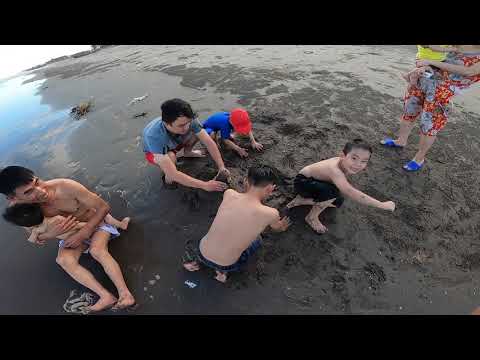The image is a detailed color photograph showcasing a family enjoying a day at a wet, muddy beach. The beach is a gradient of dark gray to light brown sand, becoming muddier closer to the blue, perfectly calm shoreline, free of any ripples. In the bottom right corner, an Asian man wearing white shorts holds a baby. Right in the center, three kids can be seen playing and building with the sand. Among them, one child with black hair wears a blue shirt and red shorts, while another, seen from the back, is in black shorts. Next to him, a boy facing the camera is only in black shorts, with mud on his arms, legs, and some on his face. Further back, another boy is wearing a blue shirt and a red cap. In the upper right corner, a woman dressed in a black, red, and yellow floral suit, with blue slippers, stands holding a baby in a yellow shirt. The serene scene is framed by black bands at the top and bottom of the photograph.